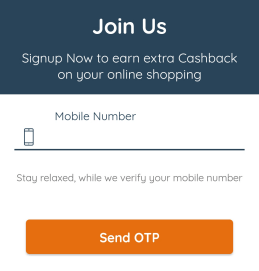This image depicts a square sign-up form divided into three distinct sections:

1. **Top Section**:
   - A vibrant blue background with a prominent white text in the center reading "Join Us".
   - Below this, in a light gray font against the blue background, it states, "Sign up now to earn extra cashback on your online shopping", though the light gray text is somewhat difficult to read due to the contrast.

2. **Middle Section**:
   - A white-background form designated for input.
   - It begins with the label "Mobile Number" followed by an icon of a phone, and a lengthy horizontal blue line, indicating the area where users should enter their phone numbers.

3. **Bottom Section**:
   - Another gray text on a white background explaining, "Stay relaxed while we verify your mobile number", again, challenging to read due to the color choice.
   - Directly below this explanation is a prominent large orange button with small white text that reads "Send OTP" (One-Time Password).

Overall, the form's purpose is clear: to recruit users for a program offering extra cashback on online shopping by collecting their mobile numbers for verification.